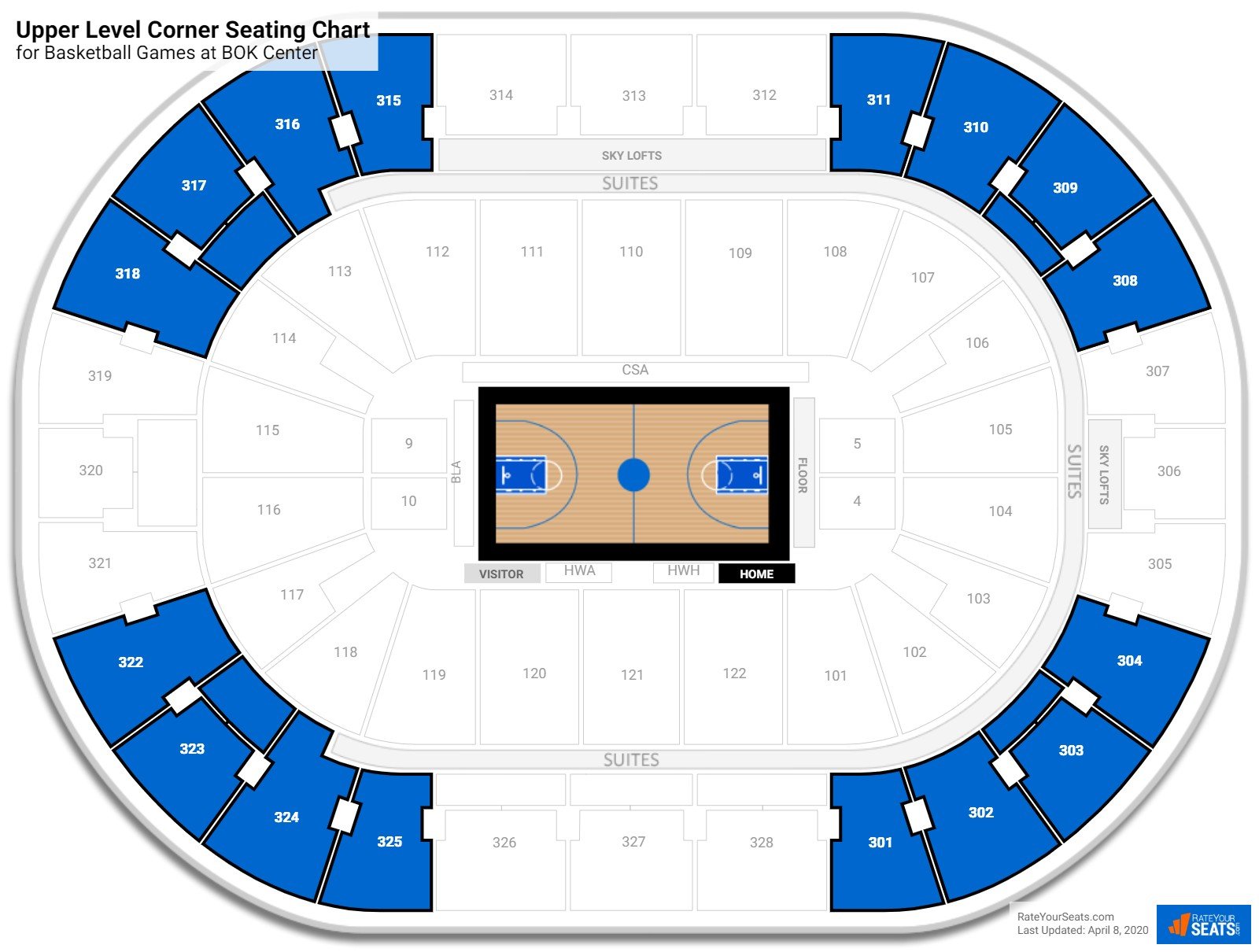The image provides comprehensive advice for selecting seats at sports venues, featuring an overhead view of a basketball arena as its primary visual. The majority of the image is occupied by this detailed graphic, which highlights the various sections of the stadium, from court-side seats to upper tiers and suites. The center of the arena is depicted as a small rectangle representing the basketball court, complete with the central circle and the rectangles marking the areas around the baskets. The left side of the court is labeled "Visitor," while the right side is marked "Home."

In the bottom right corner of the image, there is a blue rectangle housing a red logo of three bars and white text that reads "Rate Your Seats." Below this logo, the website "rateyourseats.com" is mentioned, along with a note that the information was last updated on April 8th, 2020. The purpose of this visual guide is evidently to allow users to evaluate different seating options based on factors such as visibility, proximity to the court, and overall experience, thereby aiding in the selection of the best seats within one's budget.